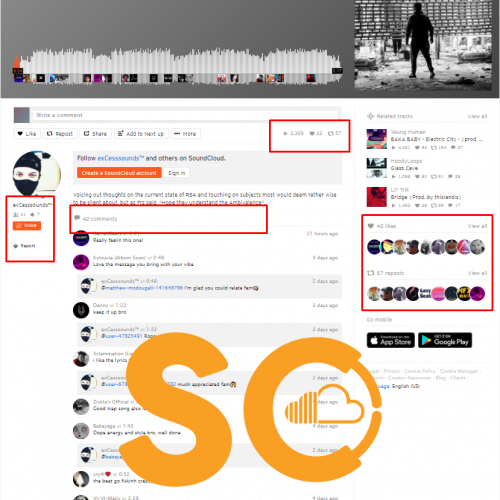The image appears to be a screenshot of a SoundCloud webpage. At the top, there is a song header displaying the length of the track, with the progress bar colored orange on the left and silver on the right, set against a dark gray background. The song's cover art, located on the right, features a person’s silhouette against a grayish background. Directly below the cover art, there is a text prompt to "Write a comment," followed by buttons labeled "Like," "Repost," "Share," and "Add to list." On the far right, some numerical data is highlighted by an orange rectangular border.

Further down, a blue "Follow" button is displayed next to the artist's name. An orange rectangle to its left contains a profile picture of an individual wearing a mask. Beneath this, there is an option to "Comment" within another orange rectangle. The comments section shows a total of 11 comments, each alternating between white and light gray backgrounds.

On the right side of the image, there are three additional song titles, presumably by the same artist. Below these titles, there is a list of profile pictures arranged in two separate rows, each surrounded by an orange square border. The very bottom of the screenshot contains buttons that link to the App Store and Google Play, both represented by black buttons.